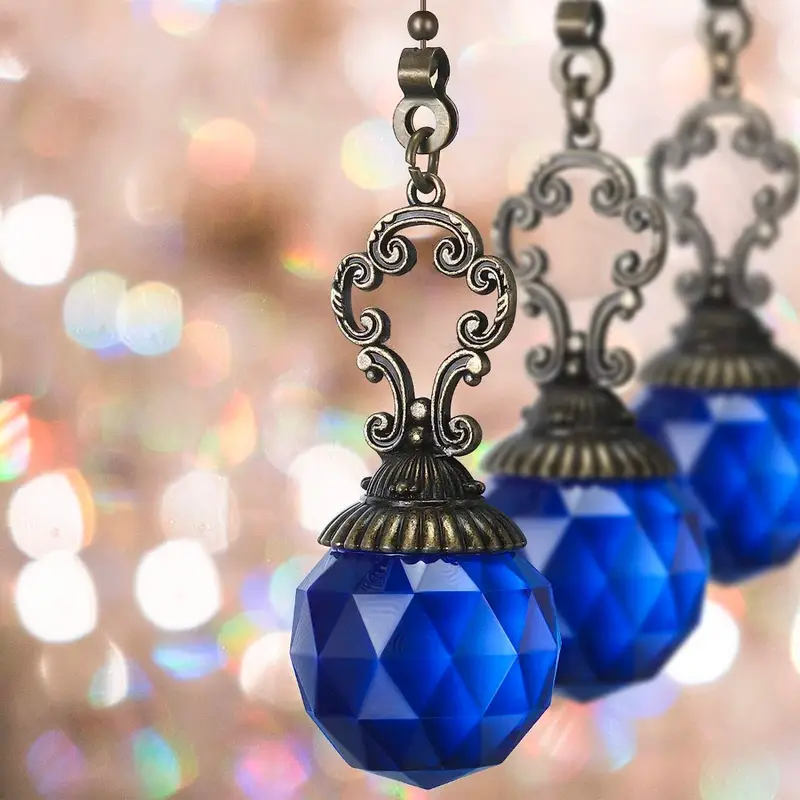The image is a zoomed-in, square shot showcasing three ornate pieces that appear to be suspended, likely from a chandelier, given the shimmering, multi-colored, unfocused lights in the background. Each piece features a deep royal blue, globular object resembling a sapphire or a disco ball, mounted directly beneath intricate brass or pewter filigree designs. These designs have a clover-like pattern with loops leading up to the suspension point. The filigree appears to be pewter or dark metal in color. The blue globes are perfectly aligned in a row, with the foremost one in clear focus, and the subsequent ones progressively blurrier. The background is filled with circular, prism-like reflections in pale hues of green, blue, pink, and white, giving the overall image a pretty and festive appearance.